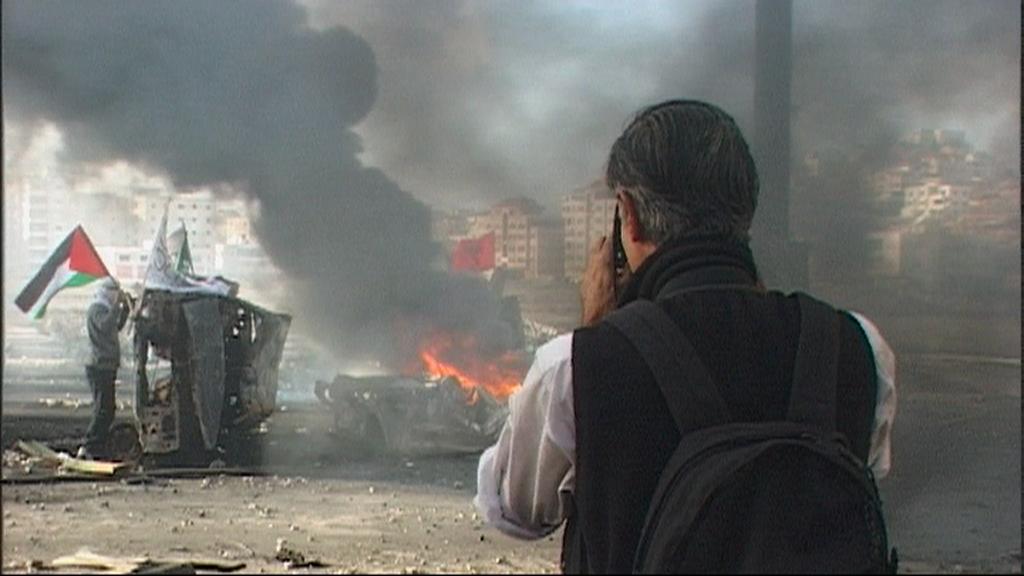In this detailed photograph, the foreground is dominated by a man seen from behind, capturing an intense scene with a camera. The photographer has salt-and-pepper hair and wears a light blue, long-sleeve shirt with the sleeves rolled up, complemented by a black, sleeveless vest and a black backpack. His stance indicates he is deeply focused on the chaotic scene ahead. 

The background depicts a war-torn cityscape obscured by thick, black smoke that billows from a burning automobile on the right side of the image. Just to the left of this vehicle sits another car, already burned out, suggesting recent explosions or severe conflict. 

Amidst the destruction stands a man on the left side of the photo, identifiable by his white turban and mask that only reveals his eyes. He clutches a Palestinian flag, notably characterized by horizontal stripes of black, white, and green, with a red triangle extending from the flag's spine. Two additional flags lean on the wrecked car beside him. The ground beneath is strewn with dirt and rocks, completing the grim tableau of devastation. Tall buildings can be faintly seen in the background, their visibility compromised by the pervasive smoke, adding depth to the scene's atmosphere of turmoil and destruction.